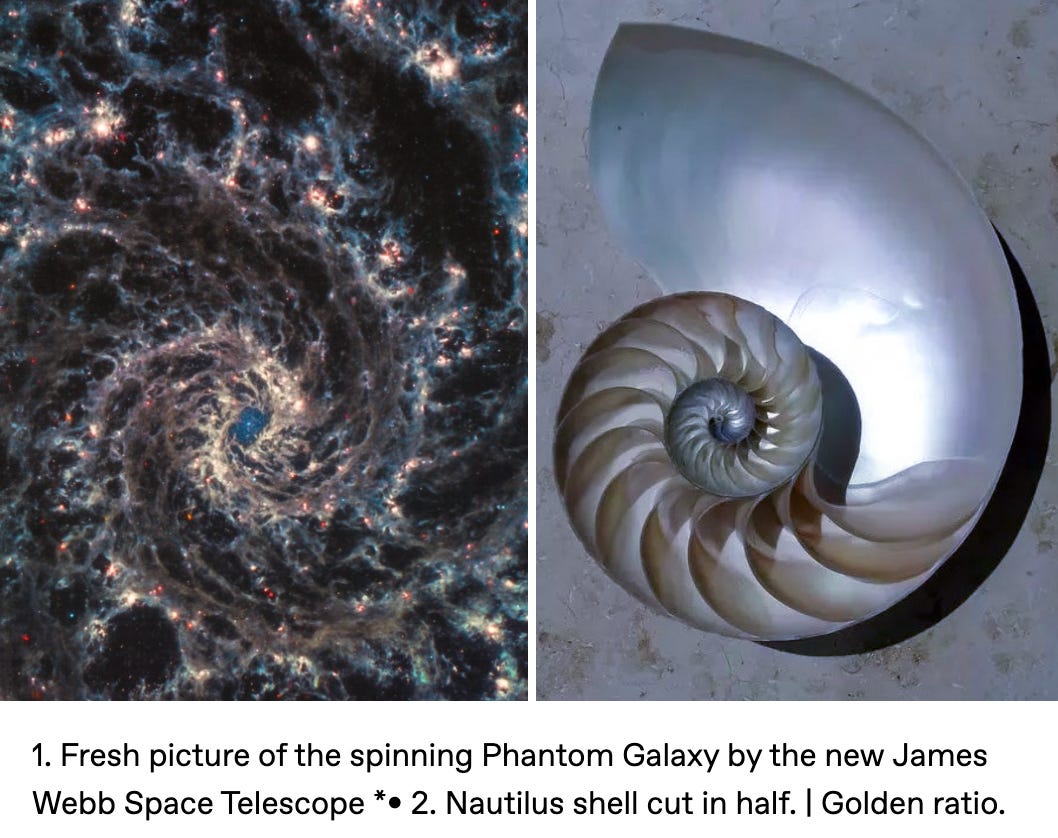This split-image comparison showcases the striking similarities between the cosmic and natural worlds. On the left, a fresh capture of the spinning Phantom Galaxy, taken by the James Webb Space Telescope, reveals intricate swirls of gray, light blue, and pink nebulae, punctuated by glimmers of red and pink stars. The dark, almost black background accentuates its corkscrew structure, reminiscent of the Milky Way. On the right, a nautilus shell, meticulously cut in half to expose its inner spirals, mirrors this celestial pattern with its smooth, reflective surface and tan designs spiraling into the curve. Both images highlight the golden ratio, underscoring the fascinating parallels between the universe's grandeur and nature's intricate designs. The nautilus shell rests on a marble table with a complementary swirled effect, and a thin white line divides the two images. Beneath the pictures, white text reads: "1. Fresh picture of the spinning Phantom Galaxy by the new James Webb Space Telescope. 2. Nautilus shell cut in half, golden ratio." The reflective glare on the inner shell adds a subtle, luminous touch to the natural marvel, enhancing the visual correlation between the two awe-inspiring subjects.